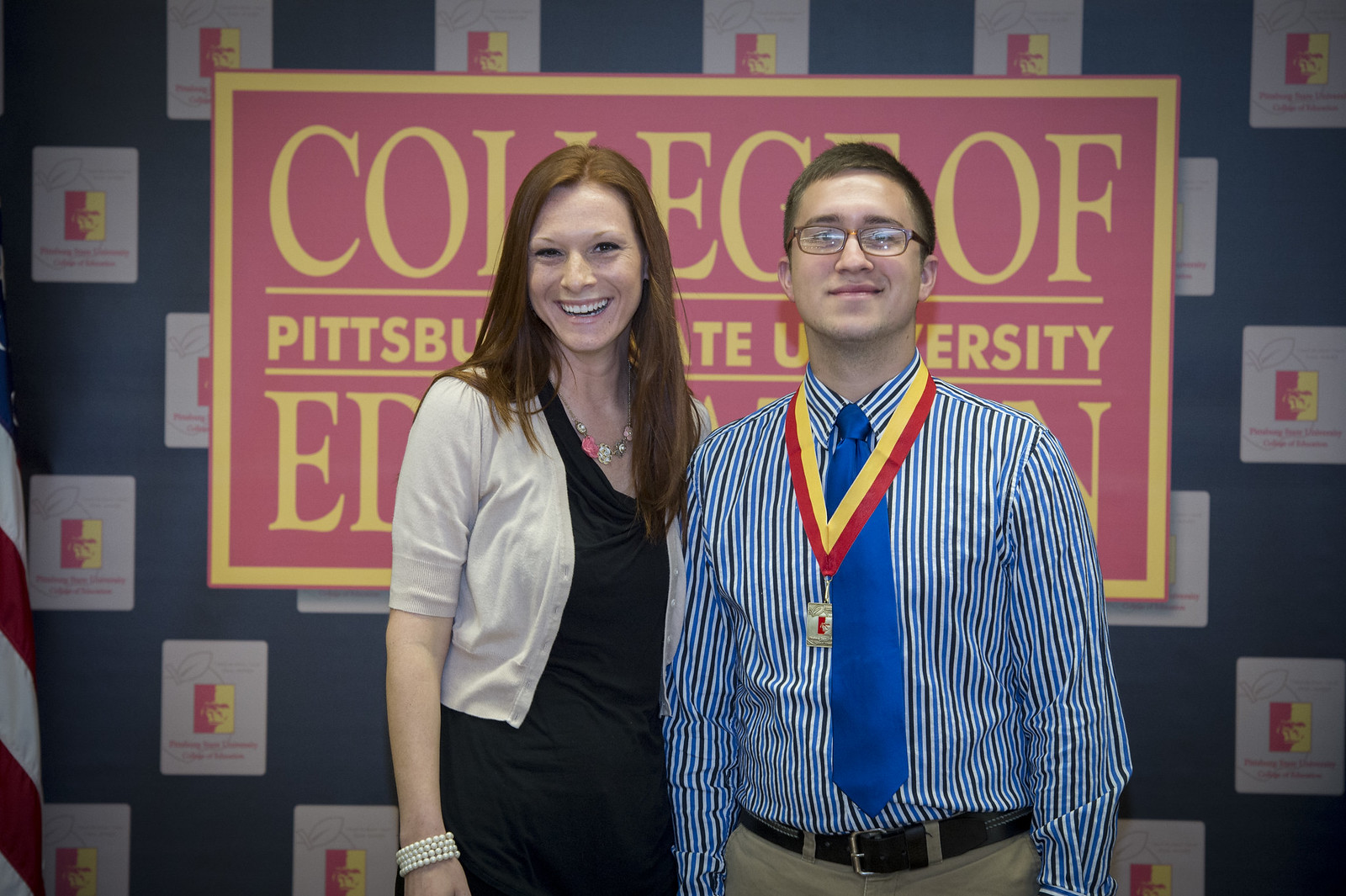In the photo, two individuals stand side by side against a vibrant and colorful backdrop. On the left is a woman with straight brown hair, wearing a white sweater over a black dress, accessorized with jewelry including a bracelet and a necklace. She is beaming a broad smile. Next to her is a young man of similar height, sporting short brown hair and glasses. He's wearing a blue and brown striped shirt paired with a long blue tie, and he's smirking subtly. The young man also has a yellow and red medal around his neck. Behind them, partially blocked by their presence, is a pink and yellow framed banner with the text "College of Pittsburgh State University" and additional unreadable text below. The backdrop includes a red and yellow sign, a blue wall with a gray box, and an American flag, enhancing the collegiate and ceremonial atmosphere.